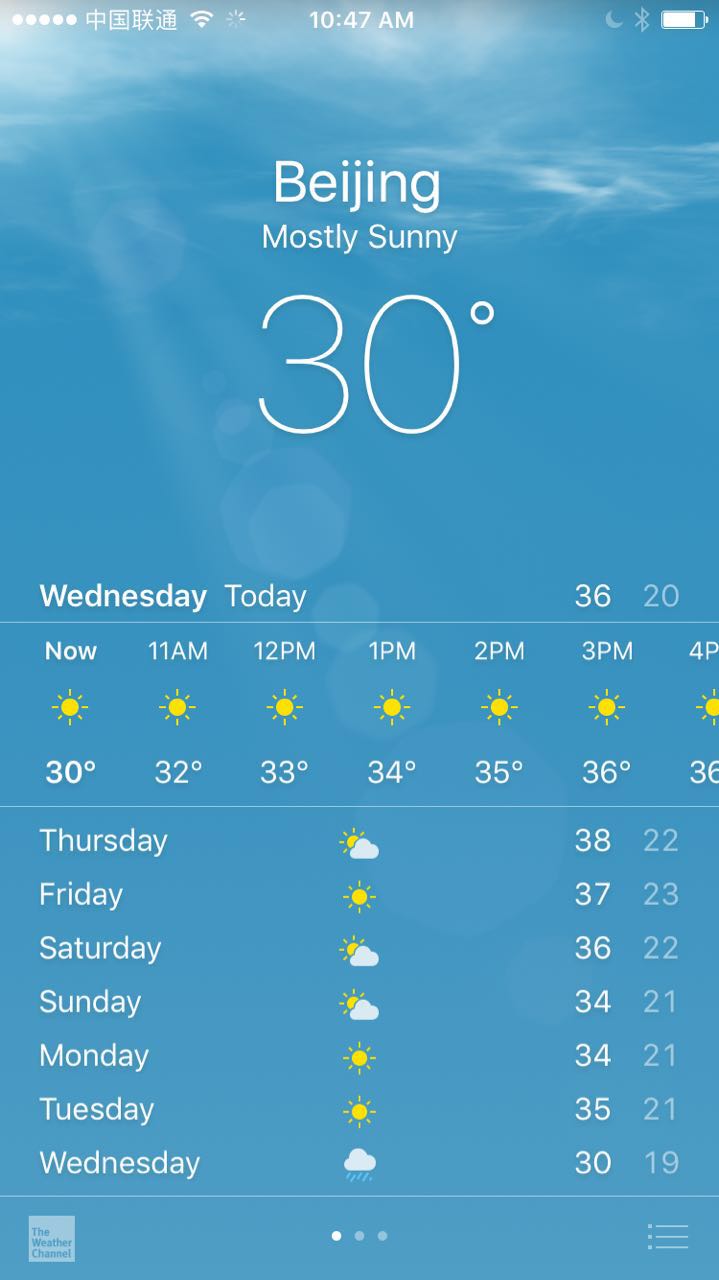The image showcases a detailed view of a smartphone screen. In the top left corner, Chinese characters are visible, accompanied by icons for Wi-Fi, Bluetooth, the time (10:47 AM), and a battery indicator. Dominating the center of the screen is a weather forecast for Beijing, indicating mostly sunny conditions with a current temperature of 30°C. The background features a serene light blue sky with a few wispy clouds.

Below the weather forecast, there's a detailed hourly temperature projection for the day, starting at 30°C at 10:47 AM, and gradually increasing: 32°C at 11 AM, 33°C at 12 PM, peaking at 36°C by 3 PM, and so on. Additionally, there is a weekly forecast with predicted temperatures: 38°C on Thursday, 37°C on Friday, 36°C on Saturday, 34°C on Sunday and Monday, 35°C on Tuesday, and finally cooling down to 30°C on the following Wednesday.